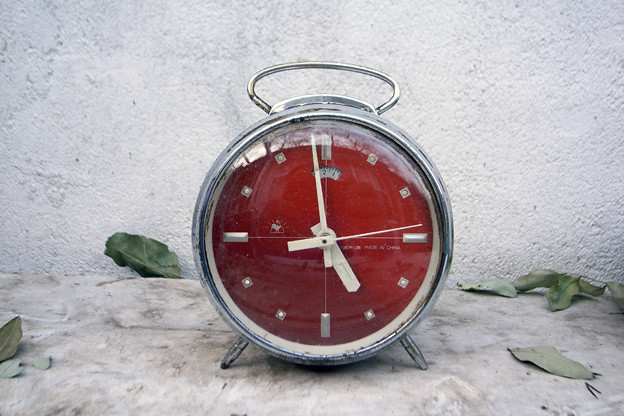This photograph features a vintage, red, steel alarm clock prominently situated in the foreground against a textured granite wall. The clock's round face is protected by a domed glass cover and distinctly lacks traditional numbers, instead displaying square markers at each hour position. The time indicated is approximately 4:57 and 13 seconds. Surrounding the alarm clock are six dried green leaves scattered on the surface it rests on, adding a touch of natural decay. The combination of the timeless design of the clock and the rustic backdrop suggests an ambiance of aged elegance.